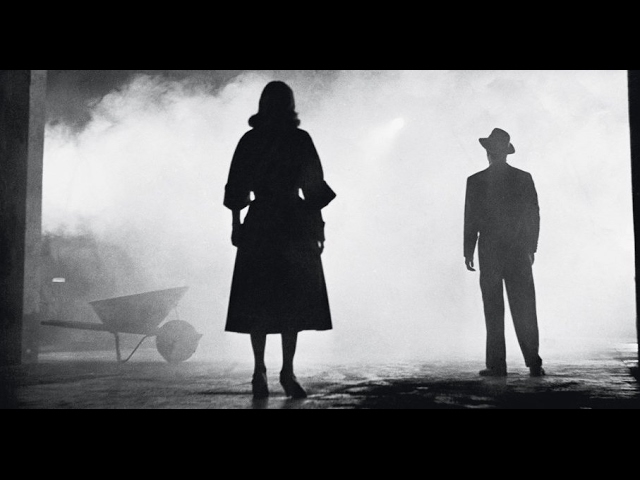In this striking black-and-white image, we see the silhouettes of a man and a woman enveloped in a dense cloud of smoke or fog, creating a dramatic and mysterious atmosphere reminiscent of a classic movie scene. The woman stands slightly left of center, adorned in a dress that flares out at the cuffs and reaches below her knees. Her hair, styled in soft curls, cascades to her shoulders as her arms hang down to her hips. She wears high heels, adding to her elegant stance. To the right of her stands a man, his silhouette distinguished by a suit and a wide-brimmed hat, tilted sideways. His legs are slightly apart, with one leg bent, giving him a poised yet casual demeanor as he faces the woman. 

In the foreground lies a wheelbarrow, partially obscured by the smoke. The wheelbarrow's tire faces towards the right, supported by triangular brackets that add to the industrial feel of the setting. The smoke, originating from the left side, grows denser as it drifts right, where it meets a concrete pillar and a wet, possibly rain-slicked concrete ground. The scene has an aura of intrigue, heightened by the silhouettes and the ethereal fog that obscures further details.